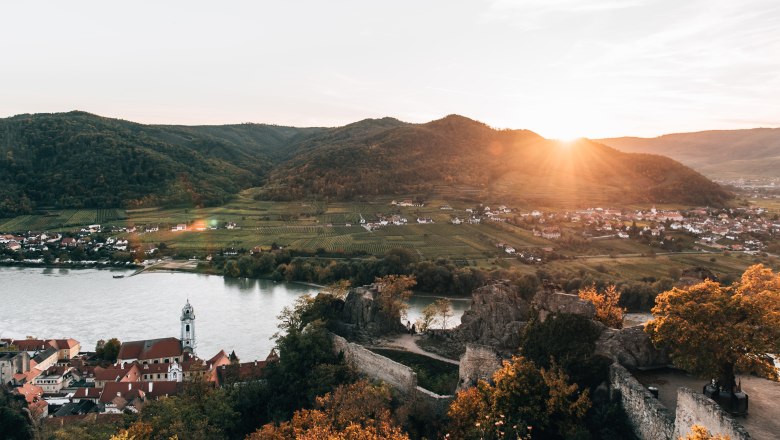This stunning aerial photograph presents a sweeping landscape, captured with professional precision from a high vantage point. At the top of the image, an overcast sky transitions to a vivid sunset, with rays of sun piercing through clouds to bathe the scenery below in a warm glow. Dominating the horizon are lush green and gray mountains blanketed in dense forests, giving way to a serene, sprawling valley below.

In the foreground of this autumnal scene, trees are tinged with vibrant hues of yellow, orange, and dark red. Nestled among the foliage are numerous small buildings, mostly white with clay-colored or brown roofs, including distinctive three or four-story structures that might be churches. On the right-hand side, there is a stone structure, possibly an overlook, peeking through the trees.

A large body of water, either a lake or an expansive pond, sits at the center of the image, bordered by these quaint buildings. Further beyond the water, additional clusters of buildings and open green fields can be seen, creating a picturesque patchwork. The overall impression is one of tranquil beauty, capturing both the natural splendor and the quaint charm of human habitation, making this image worthy of being framed and displayed in any museum or fine living room.